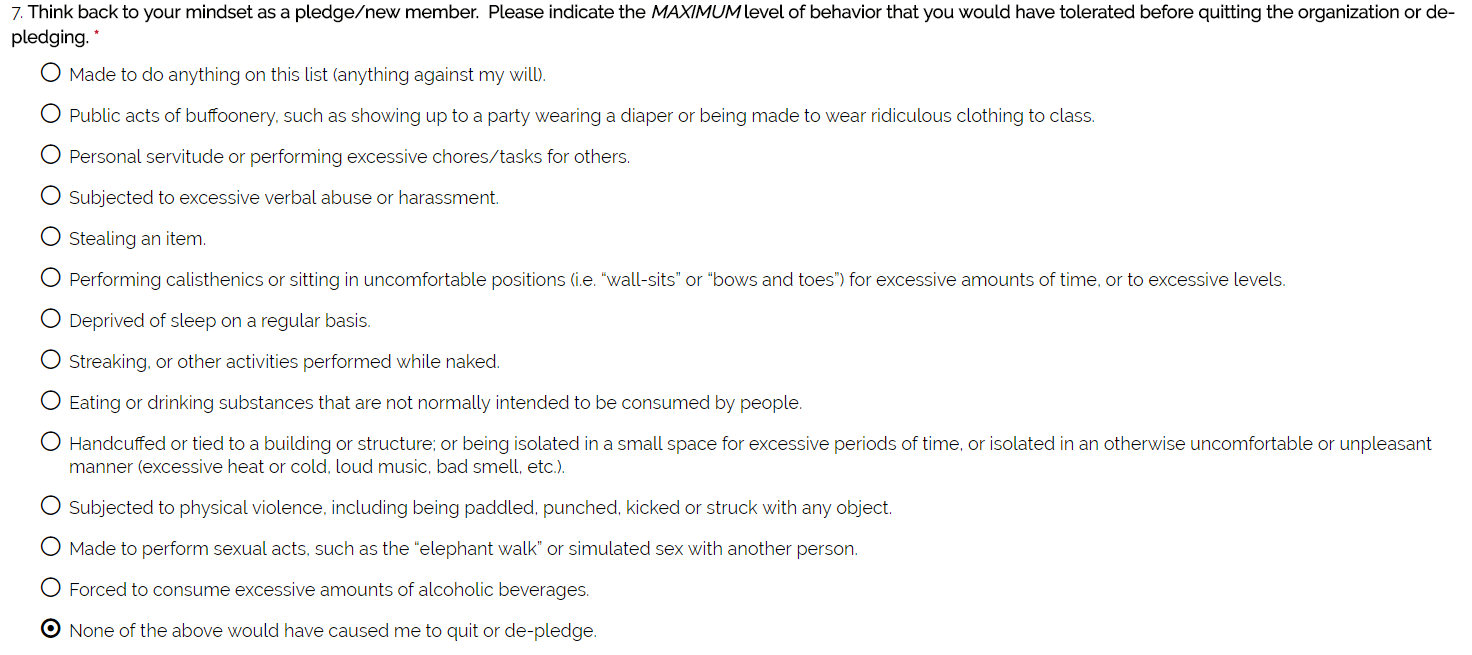Here is a cleaned-up and detailed caption for the described image:

---

This image features a scanned or screenshot of a multiple-choice question from a survey or form, likely related to college pledges. At the top, in bold print, it reads: "7. Think back to your mindset as a pledged new member. Please include the maximum level of behavior that you would have tolerated before quitting the organization or de-pledging." The text appears slightly blurry and is printed with inconsistent ink levels, making it difficult to read. Some words are darker, while others are faded, indicative of a printer running low on ink.

The form contains several bullet points, each accompanied by a circle for respondents to check their answer. The options list various behaviors, and the one that is checked reads: "None of the above would have caused me to quit or de-pledge."

The other bullet points detail specific types of unacceptable behaviors, including:
- Being made to do anything on the list against one's will.
- Engaging in public acts of buffoonery, such as attending a party wearing a diaper or wearing ridiculous clothing to class.
- Performing personal servitude or excessive chores/tasks for others.
- Being subjected to excessive verbal abuse or harassment.
- Stealing items.
- Performing calisthenics in uncomfortable positions.
- Being deprived of sleep on a regular basis.

The form's overall condition suggests it is used for assessing tolerance levels of different behaviors during the membership pledging process for a college organization.